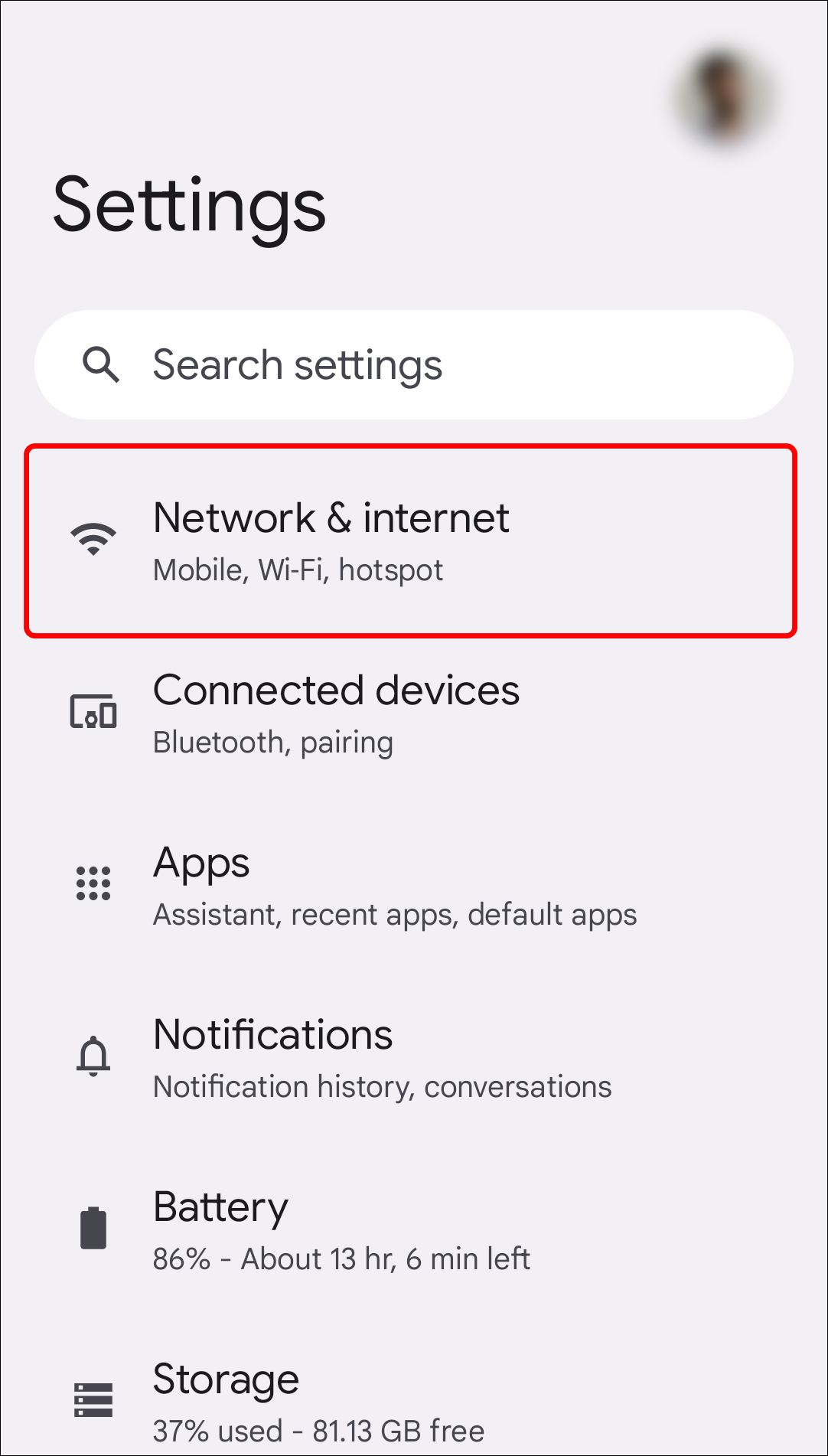This vertical mobile screenshot features a sleek, thin grayish border framing a light gray background. In the top-right corner, there is a heavily blurred circular thumbnail that suggests the silhouette of a dark-skinned individual, possibly a male. On the left side of the screen, the word "Settings" is prominently displayed in bold, black text. Directly below this, a white search bar contains the placeholder text "Search settings."

The first section lists "Network & internet," with the options for "Mobile" and "Wi-Fi hotspot," all encased in a red rectangle accompanied by a Wi-Fi icon. The next section, "Connected devices," features options for "Bluetooth pairing," paired with an icon that depicts a mobile device and a screen. Following this, the "Apps" section includes options for "Assistant," "Recent apps," and "Default apps," represented by a three-by-three grid of black dots.

The "Notifications" section details options for "Notification history" and "Conversations," denoted by a bell icon. The "Battery" section shows the battery level at 86%, with an estimated 13 hours and 6 minutes of usage left, and is illustrated by a black battery icon. Lastly, the "Storage" section indicates that 37% of storage is used, leaving 81.13 GB free.